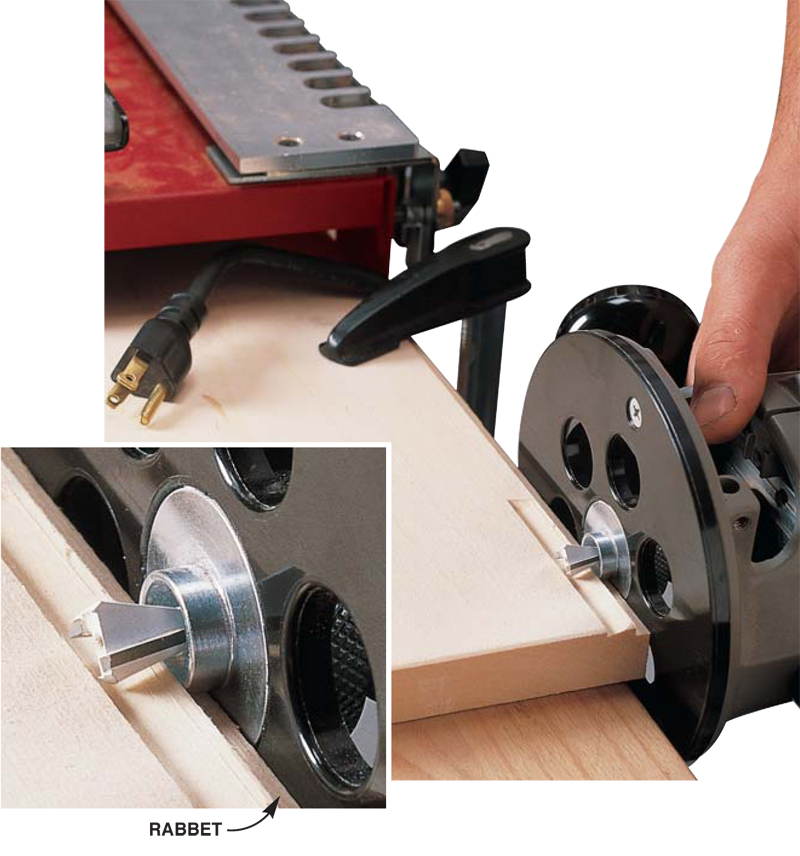The image showcases a detailed view of a woodworking process involving machinery. Central to the scene is a piece of pine wood, rectangular in shape, with a person's hand guiding a specialized tool. This tool, labeled as a "Rabbet," features a distinctive circular black cutout and a silver metal component. The hand appears to drag the black circular piece along the wood, which results in a deep incision made by the silver chisel-like part of the tool. A black arrow points towards the "Rabbet" label, emphasizing its function. On the lower left of the image, there is black text that reads "RABBET". The wood, possibly part of a larger construction project like a house, bears the marks of the tool's impressions. Additionally, the setup includes a red painted block of wood, a plug with a gold end, and a small black object, hinting at the electrical nature of the tool. The hand is seen positioning everything in place, ensuring the tool moves correctly along the groove of the wood. This detailed capture highlights both the precision and intricacy involved in the woodworking technique.